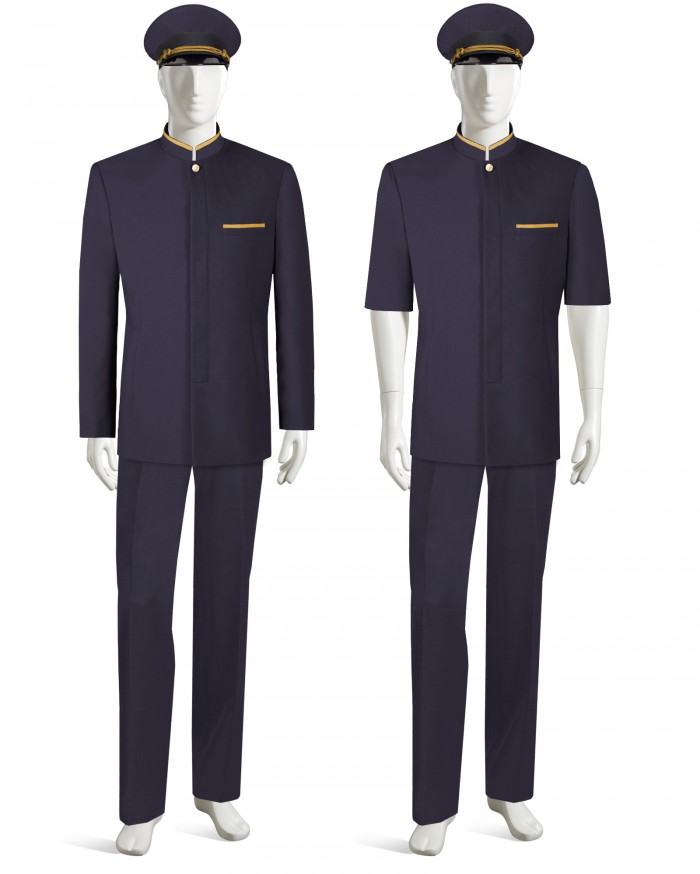The image shows two white, adult-sized, male mannequins standing side-by-side against a white background. They are dressed in deep navy blue uniforms, resembling conductor outfits. Each outfit includes matching suit pants and a button-up top with a raised collar. Both tops feature gold trims at the collar's edge and the pocket's top, accompanied by a gold button below the collar. The only difference between the outfits is that one is long-sleeved (on the left) and the other is short-sleeved (on the right). Each mannequin also sports a matching navy cap with a black brim and a gold band. The mannequins stand straight with arms at their sides, showcasing the distinct, detailed attire.